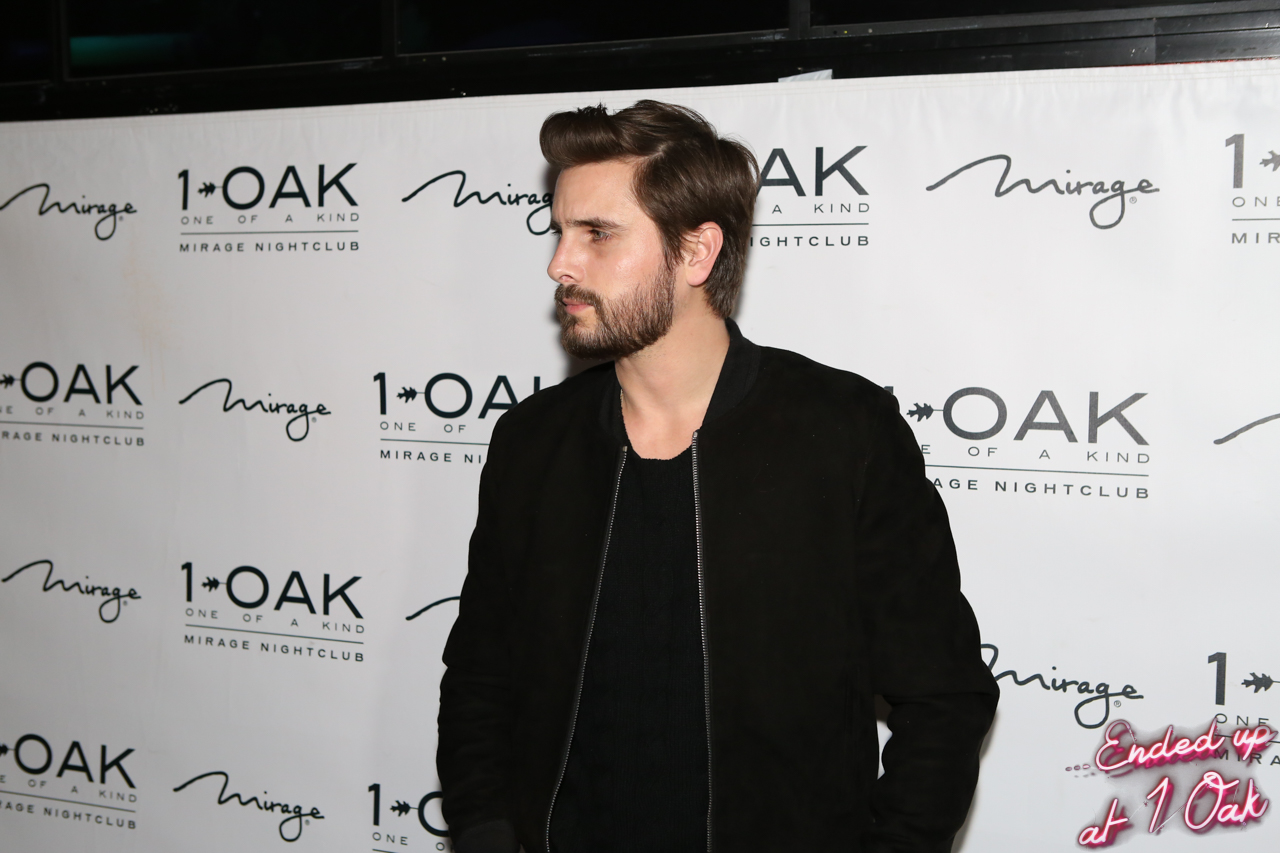A young man, likely in his thirties, is captured standing in front of a large white banner adorned with alternating logos that read "Mirage" and "One Oak" in a patterned fashion. The background is predominantly black in the upper half, giving a nighttime ambiance. The man, sporting medium-length brown hair parted on the left and combed over, has a full mustache and beard. He is dressed in a black, open zip-up jacket with white trim over a black round-neck shirt. His hands appear to be in his pockets, and he stands at a three-quarter angle, looking off to the left. In the bottom right corner of the photograph, white lettering shadowed in black, resembling a neon sign, reads "ended up at One Oak." This snapshot seems to be taken at a red-carpet event hosted by Mirage Nightclub.